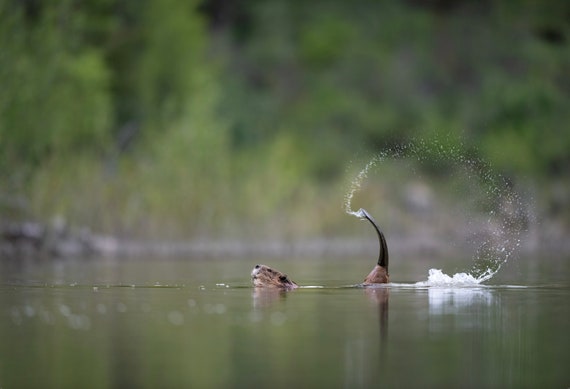In this photograph, a brown beaver is the focal point, swimming in a calm lake with its distinctive flat tail dramatically arcing out of the water, flinging droplets to the right. The beaver's head is partially submerged, revealing its black eye and face while its body remains mostly beneath the water's surface. The water is disturbed and white where the tail emerged. The lake reflects a slightly brownish tinge, and the serene scene is accentuated by a backdrop of blurry green trees. The background suggests daytime, with hints of rocky terrain along the riverbank, contributing to the natural and tranquil setting.